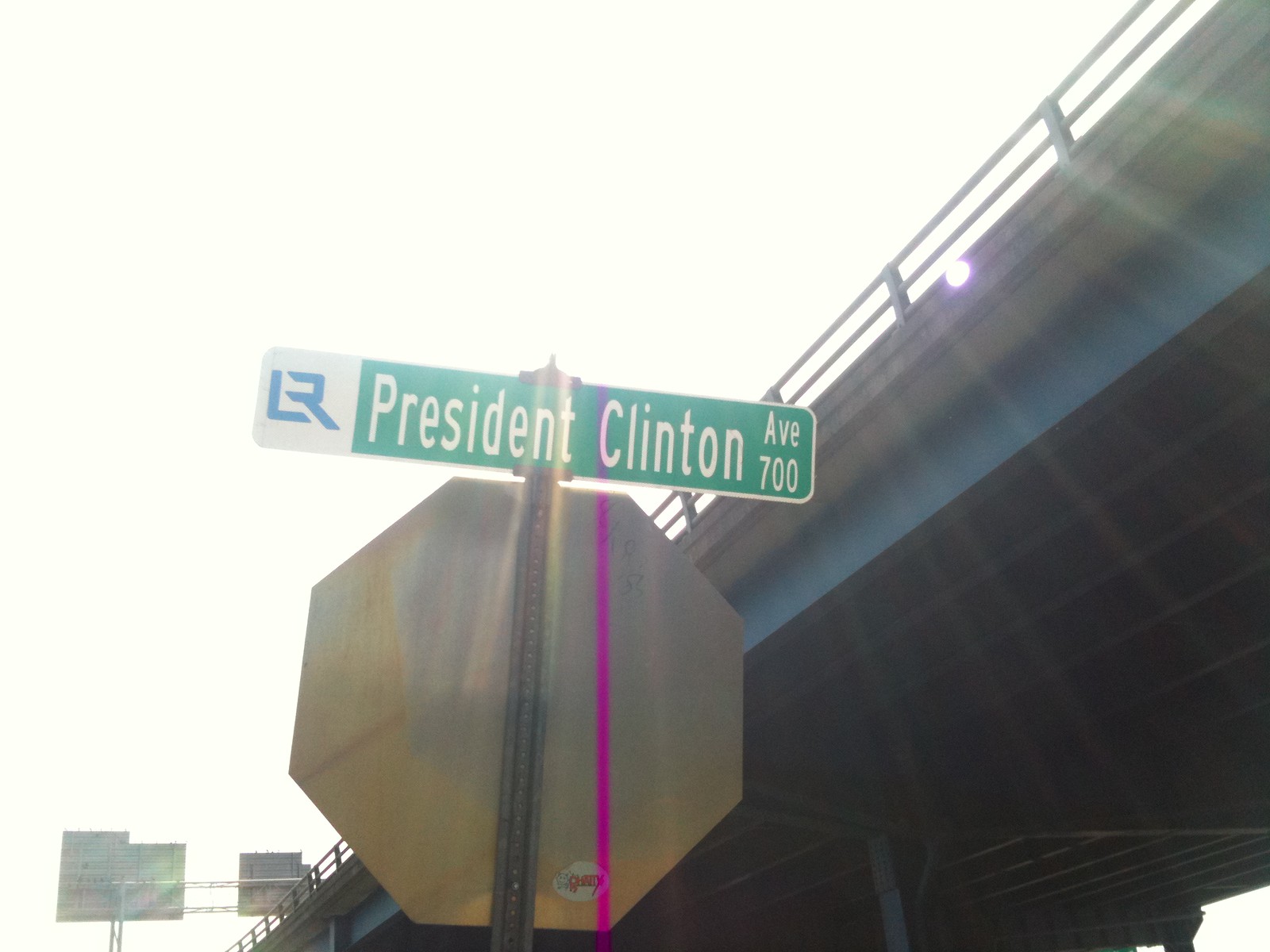This image captures a green street sign with white lettering that reads "President Clinton Avenue," indicating the 700 block. The sign, also featuring a white background on the left with a blue symbol resembling the letters "LR," is mounted atop a metal pole, positioned above and behind a stop sign. Both signs are situated beneath an overpass bridge, detailed by the overexposed, white sky. In the background, the rear sides of highway signs are visible, extending across the road. This urban scene is taken from an angle that showcases the structural elements of the stop sign, the pole, and the overhead bridge infrastructure.